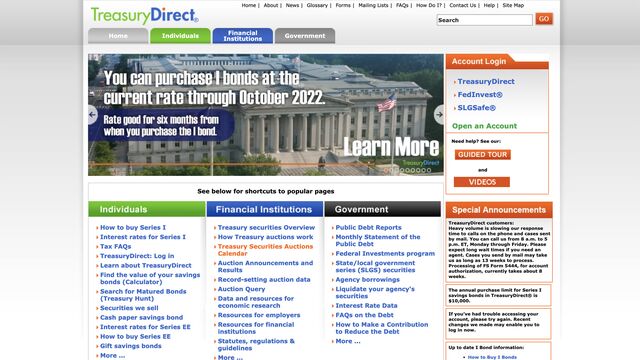The image depicts the Treasury Direct website. At the very top of the homepage, several navigation options are visible, including Home, About, News, Glossary, Forms, Mailing Lists, Facts, How Do I…, Contact Us, Help, and Sitemap. Beneath these, there are categorized tabs labeled Home, Individuals, Financial Institutions, and Government. On the right-hand side, users have quick access to Account Login, Open an Account, Guided Tour, and Videos.

The website prominently features a headline announcing the current rate for purchasing iBonds, valid through October 2022, and specifies that the rate is good for six months from the purchase date. A "Learn More" link is also available for additional information.

Lower on the page, four highlighted columns provide shortcuts to popular sections: Individuals, Financial Institutions, Government, and Special Announcements. Each column aims to offer streamlined navigation for different user categories.

Specifically, within the Financial Institutions column, there is an imminent action suggested where the cursor appears to be hovering over or ready to click on the Treasury Security Auctions Calendar link.